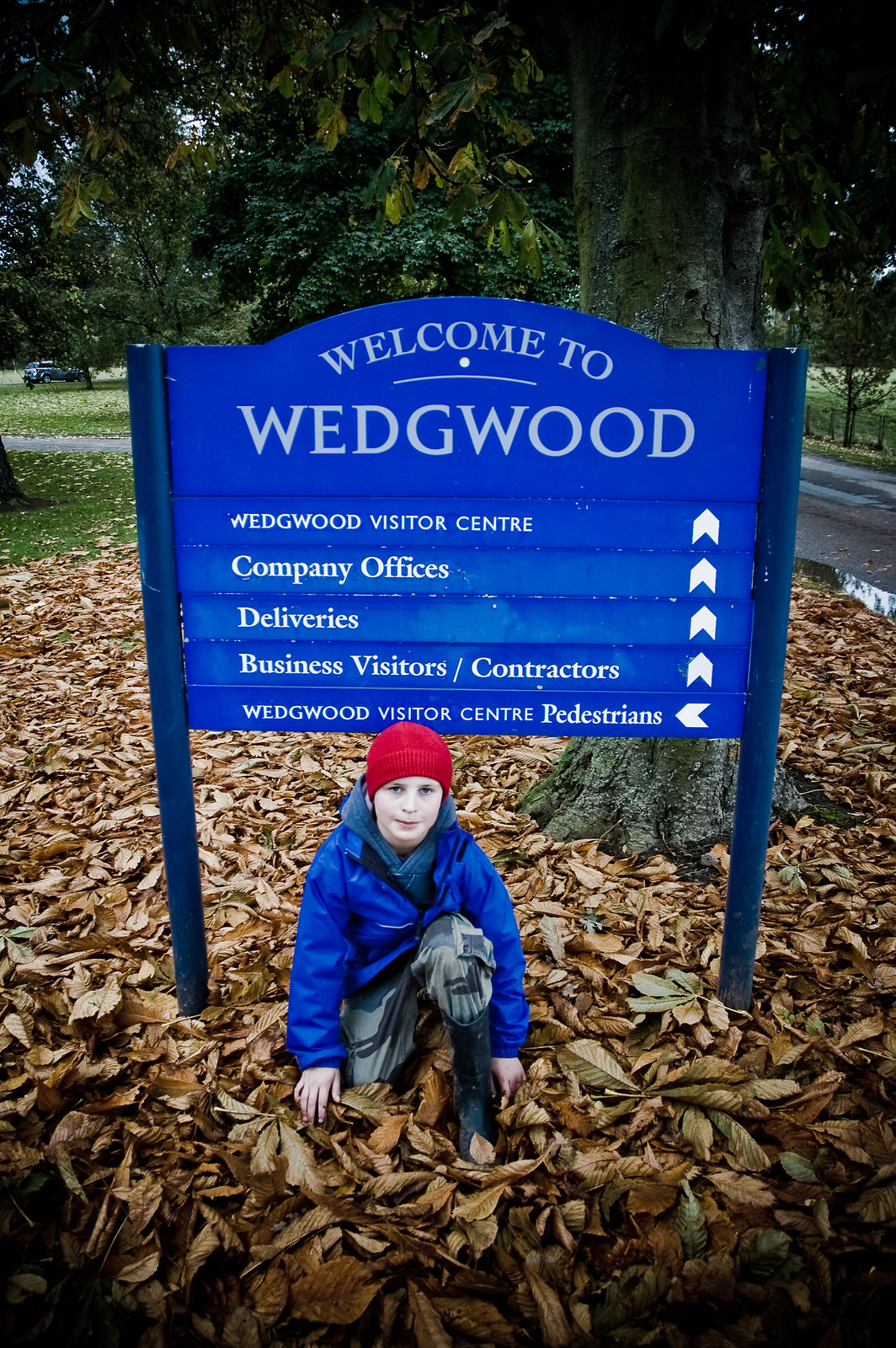A young boy, approximately 10 to 12 years old, kneels in front of a blue metal city sign that says, "Welcome to Wedgwood." The sign features white text and various directional arrows, including northward arrows for the Wedgwood Visitor Center, company offices, deliveries, and business visitors/contractors, as well as a leftward arrow for Wedgwood Visitor Center pedestrians. The scene is set in autumn, with the ground and the boy both littered with fallen brown leaves, likely from the large tree visible in the background. The grass is nearly covered by the leaves, but some patches still show through. Additional foliage and a distant park can be seen in the background. The boy is dressed in a red ski cap, a blue jacket, camouflage pants, and black rain boots, with one hand resting on the ground.